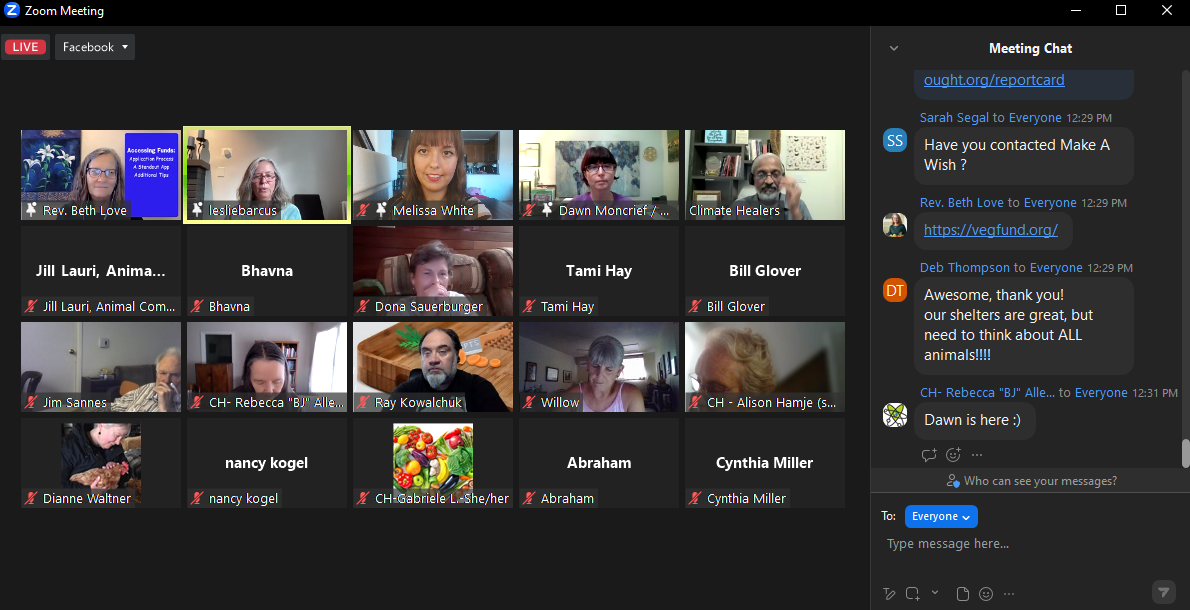At the very top left corner of the image, the words "Zoom Meeting" are displayed, accompanied by a red box containing the word "Live" and the word "Facebook" beside it. Below this, the screen is divided into multiple squares, each featuring a different participant.

The square outlined in green highlights a woman with shoulder-length gray hair and glasses. Next to her on the right is a smiling woman with short brown hair. Adjacent to her, another woman with dark brown hair, glasses, and a purple shirt appears. On the far right of the row is a man sporting gray hair, a gray beard, glasses, and a black mustache.

In the second row, there is a man sitting against a brown chair, with brown hair and his hand near his mouth.

In the third row, a man in the center is seen wearing a black shirt and having a gray beard. To his right is a woman with gray hair wearing a pink sleeveless shirt.

On the top right side of the screen, the words "Meeting Chat" are visible. Below this, in a blue circle, the letters "SS" are displayed. The chat conversation below shows a message asking, "Have you contacted Make-A-Wish?" followed by someone responding, "Awesome, thank you. Our shelters are great, but need to think about all animals."